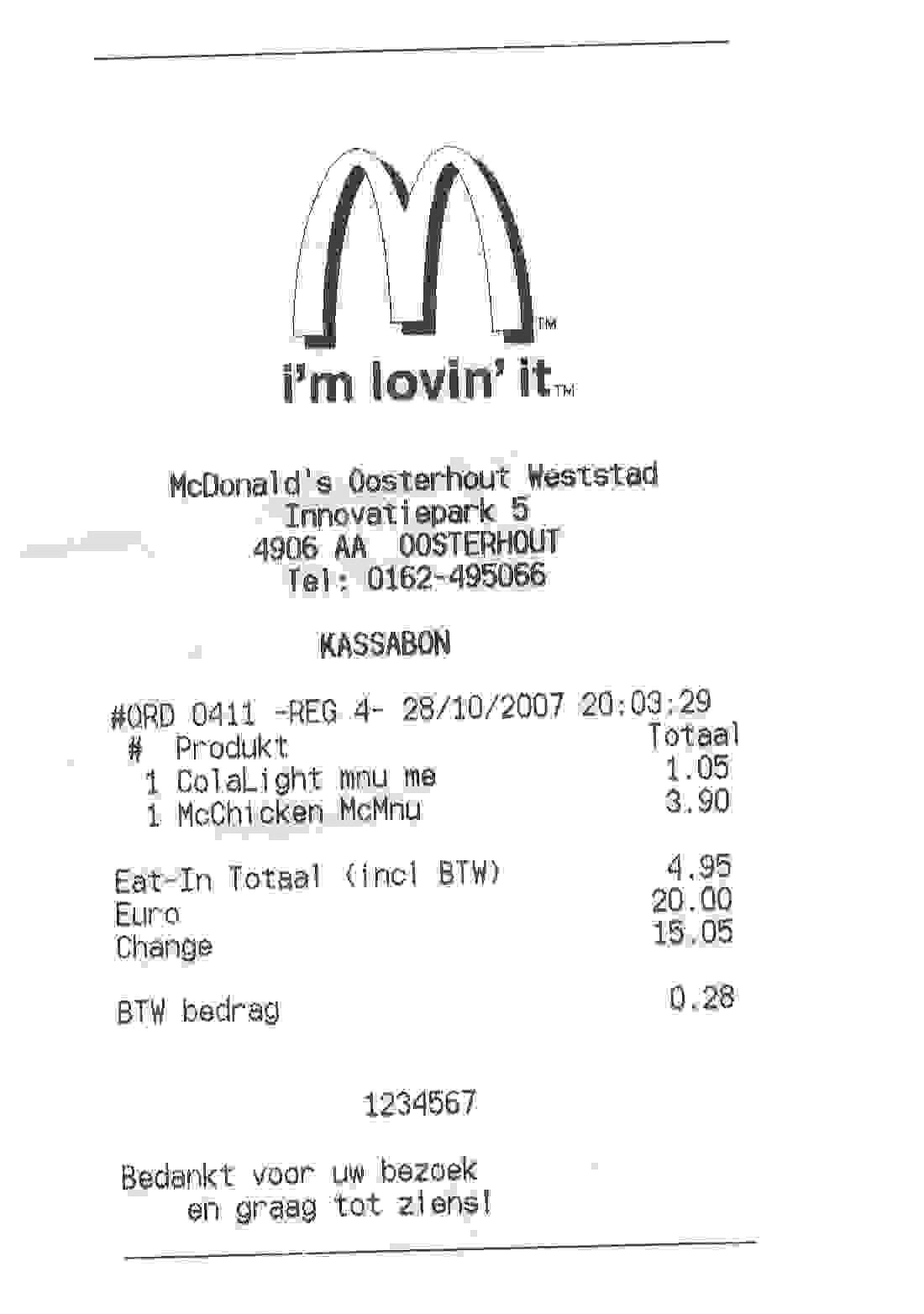This is a detailed photograph of a slightly tilted McDonald's receipt set against a white background with black print. At the top, it features the iconic McDonald's arch logo followed by the slogan, "I'm lovin' it." The receipt is from McDonald's Osterhout Weststad, located at Innovatie Park 5, 4906 AA, Osterhout. The telephone number listed is 0162-495066. 

The details of the purchase include one Cola Light priced at €1.05, and a McChicken McMenu priced at €3.90, totaling €4.95. The customer paid with a €20 note, receiving €15.05 in change. Additional details on the receipt include the text "Casabon" and a VAT (BTWBDRAG) rate of €0.28. The order number 0411 and the time and date of purchase, October 28, 2007, are also visible. Various numerical figures and text appear at the bottom, printed in a different language, and the entire receipt is bounded by thin black lines at the top and bottom.